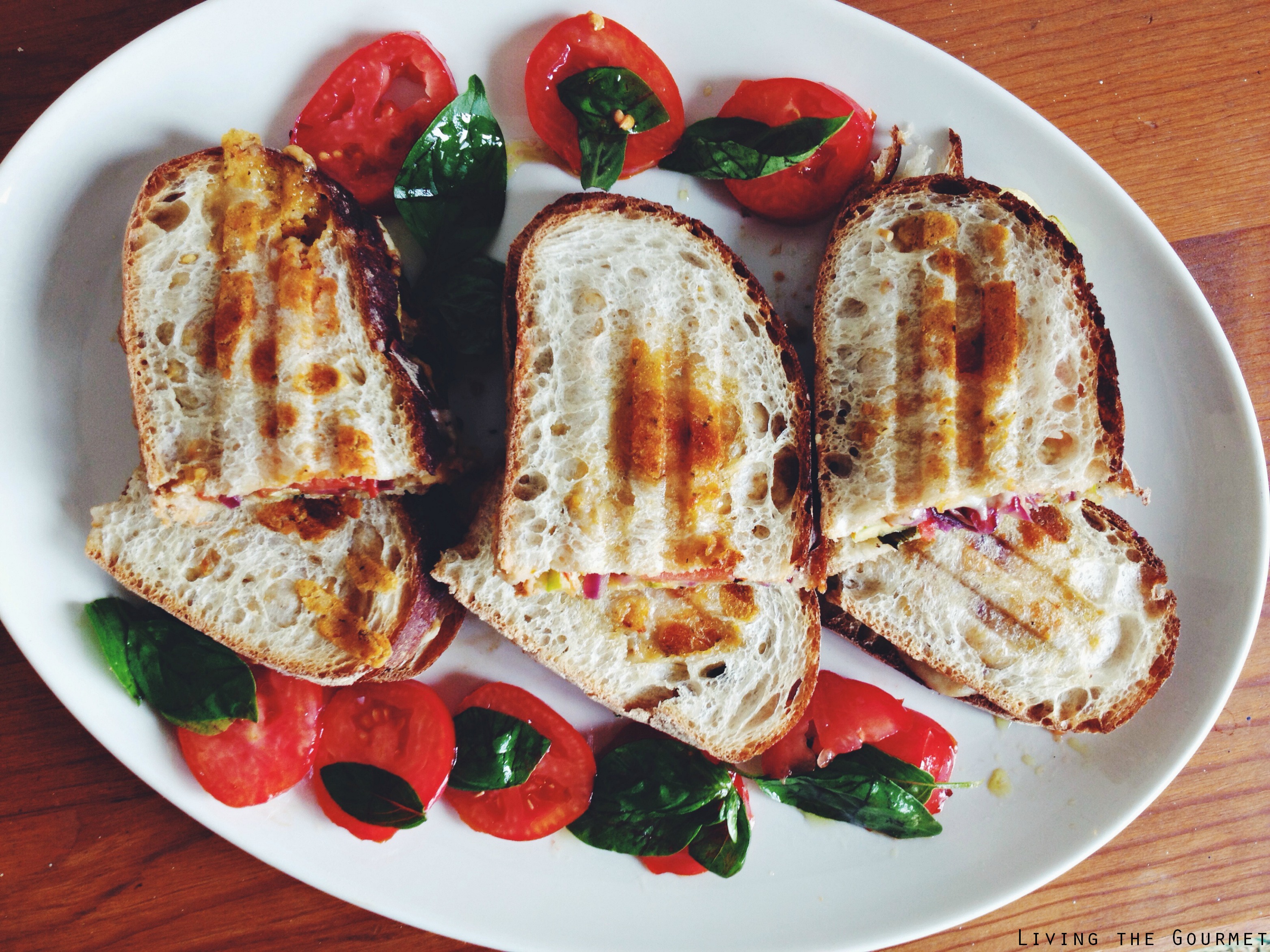The image depicts a top-down view of an indoor kitchen scene featuring a breakfast arrangement on a medium brown wooden table. Centered on the table is a large, white, oval saucer holding multiple baguette slices, characterized by their lovely brown toasted spots and dark crusts that appear almost burnt. Due to limited space, the slices are stacked atop each other, creating a layered effect. Adorning the perimeter of the plate are vibrant red cherry tomato slices, glistening with oil and complemented by fresh green basil leaves. The arrangement is presented with a decorative touch, enhancing the visual appeal. At the bottom right of the plate, small black text reads, "Living the Gourmet."